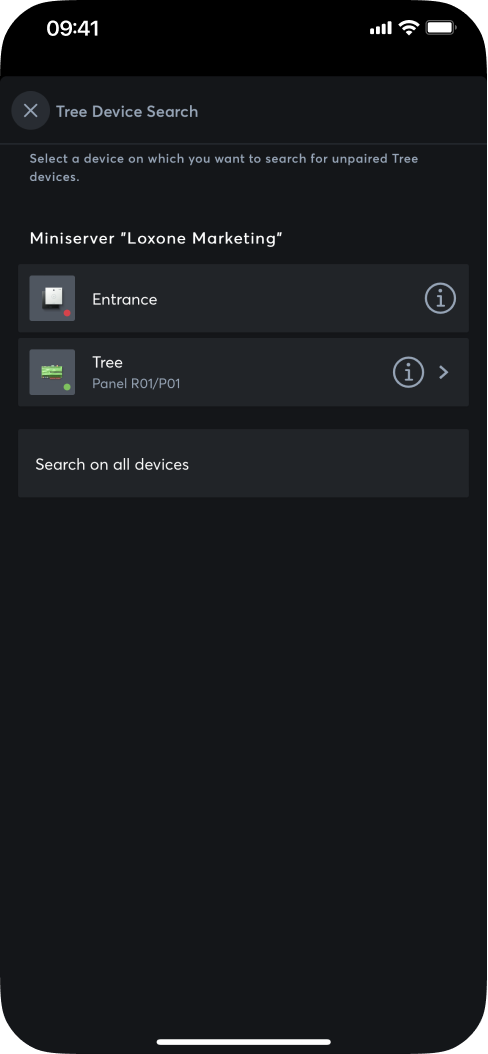The image depicts the screen of a smartphone with a black background. At the top, the screen displays the time "9:41" along with icons indicating full cellular signal, Wi-Fi connectivity, and a fully charged battery. 

Below this status bar, there is a section featuring a black or dark gray circle with a white "X" inside it, followed by the text "Tree Device Search". Just beneath, there is a line separator and a longer text that reads, "To select a device on which you want to search for unpaired tree devices."

The next section features a label "Lexicon Marketing" enclosed within quotation marks, followed by a gray band labeled "Entrance" with an information icon (a circle with an "i" inside it) to the right side. 

Following this, another band is labeled "Tree Panel R01 / P01", also accompanied by an information icon and a right arrow symbol on the right side.

Further down, the screen has another dark gray band labeled "Search on all devices," beneath which is an empty black field that takes up about half the remaining screen space.

At the very bottom of the screen, a white line runs horizontally across the middle.

Overall, the screen is devoid of buttons on the edges, maintaining a sleek and minimalistic design with rounded corners on all four sides.